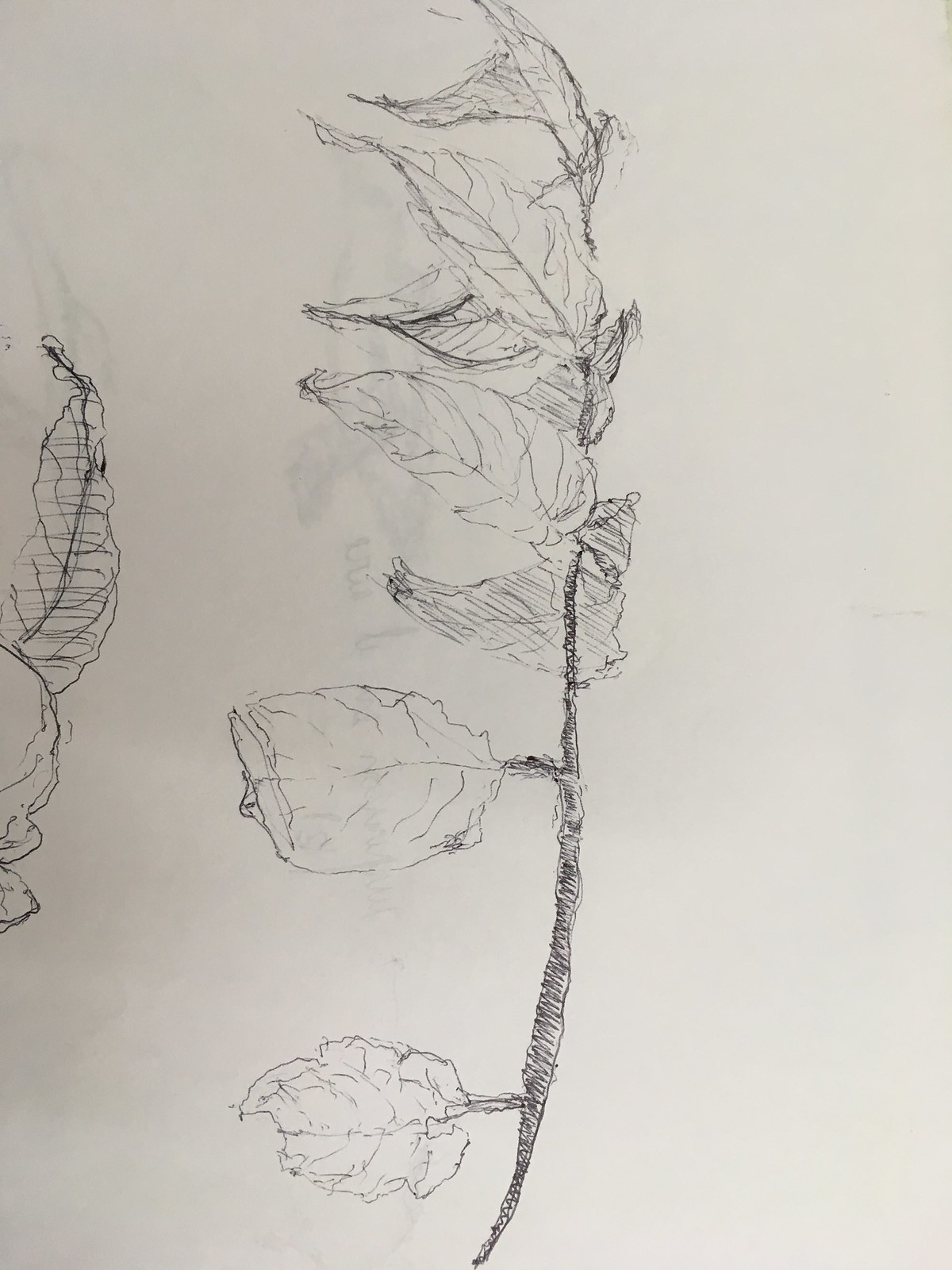The image portrays a drawing on a piece of tan-colored paper. The medium appears to be pen, evidenced by its bold and defined lines, in comparison to typical pencil shading. Central to the composition is a vertically oriented branch sketched with a wavy line texture, creating a stick-like appearance. Offshooting to the left from the lower portion of the branch are two leaves, while the top of the branch supports about six or seven additional leaves, each distinct in texture and form. The leaf at the base of the image is notably crinkled and worn, contrasted by a more orderly yet intricately curled leaf slightly above it. Each leaf is detailed with visible veins and varied shading, enhancing their naturalistic appearance.